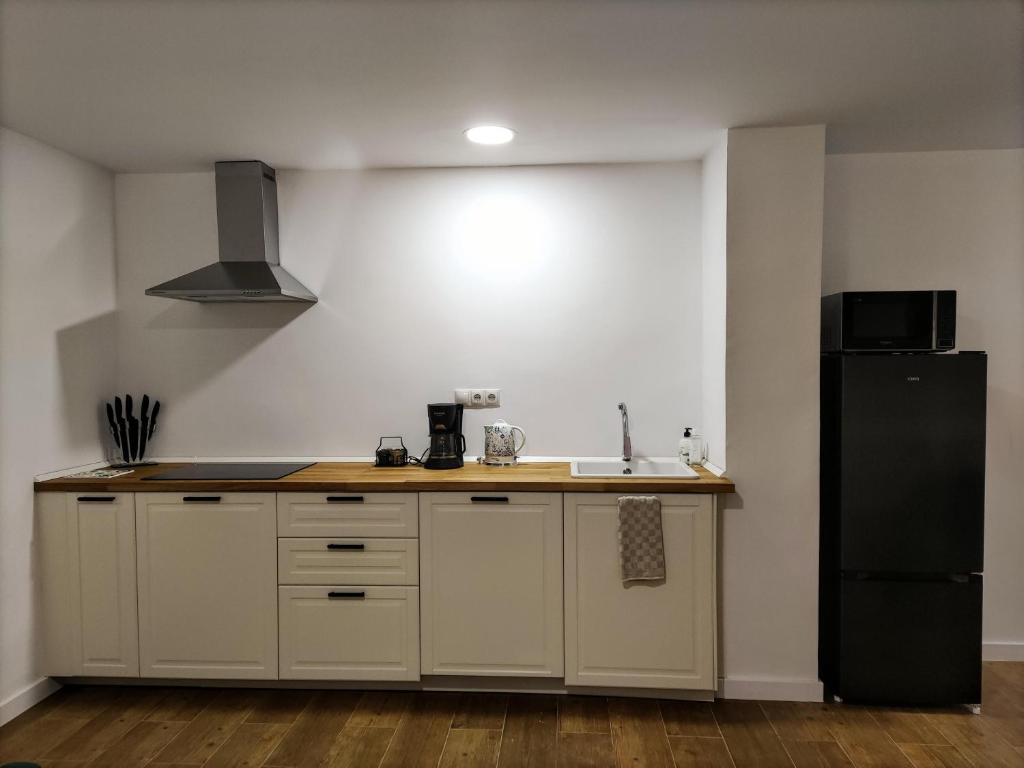The image depicts a compact kitchen, likely in an apartment or office break room, with a minimalist design characterized by its white walls and low ceiling. The kitchen features a single butcher block countertop, accompanied by cream-colored lower cabinetry with horizontal black recesses serving as handles. There's a small bar-sized square sink with a faucet and a pump bottle of soap next to it. Above the sink, a single recessed light creates a glaring reflection on the white walls, resembling a glowing sun. A stainless steel exhaust hood is mounted on the wall above a flat-surface drop-in stovetop, possibly induction. The countertop hosts a black coffee maker, an electric tea kettle, and what appears to be a knife set in a block. The floor is covered in hardwood, enhancing the warmth of the space. Next to the sink is a partition wall that separates the counter area from a small black refrigerator with a microwave perched on top.